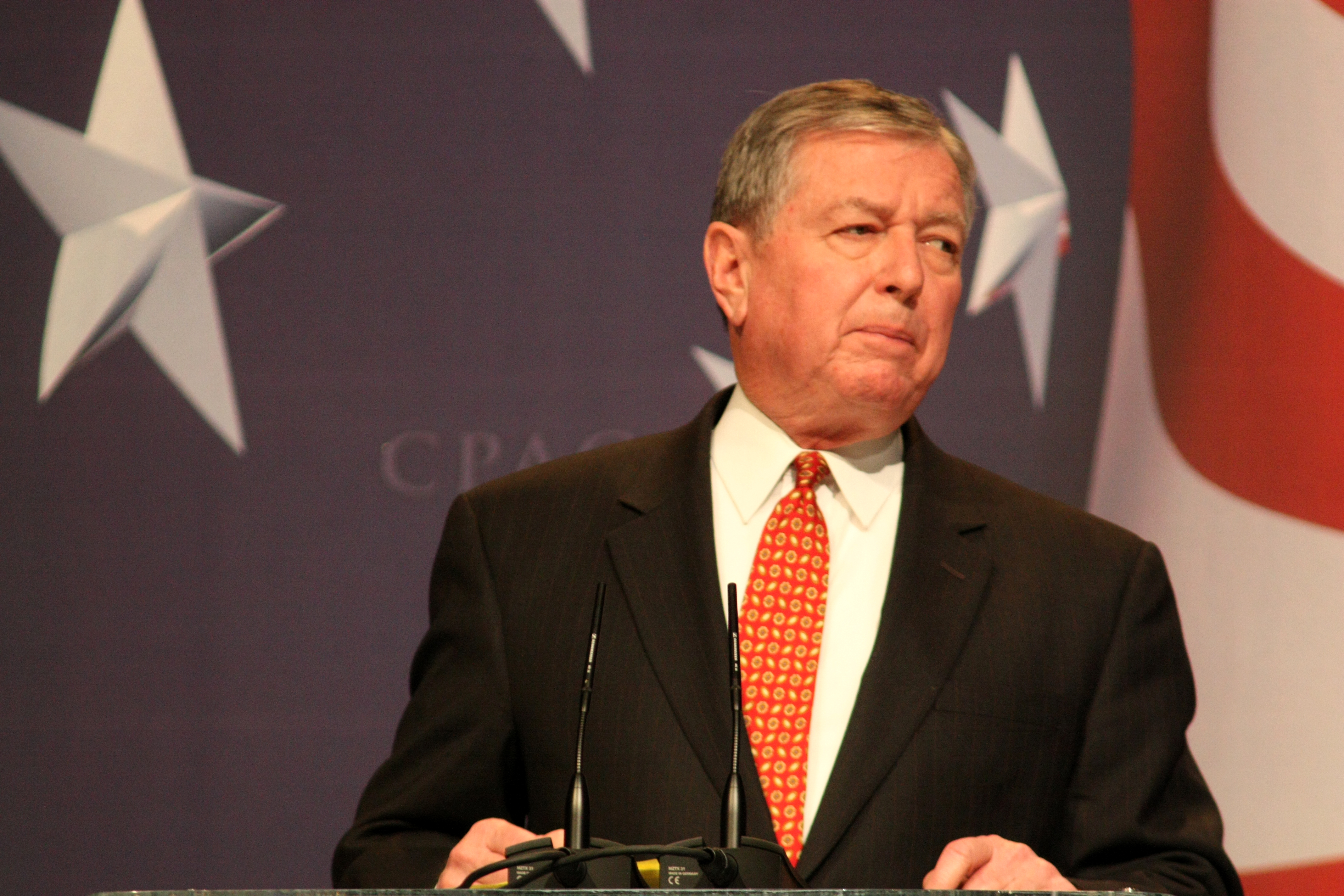In this image, we have a conservative politician standing at a podium during the Conservative Political Action Committee (CPAC) event. He is wearing a dark black suit with a white collared shirt and a red paisley tie. The politician, who has short gray and brown hair, is looking off to his left with a serious and concerned expression on his face. Behind him, the backdrop features a prominently displayed American flag with navy blue and red-and-white stripes, along with large 3D stars and the CPAC logo. His right hand is resting on the podium, which has some kind of black electronic device, possibly a modem or router, wired up in front of him. The setting underscores his commitment and the formal tone of the event.